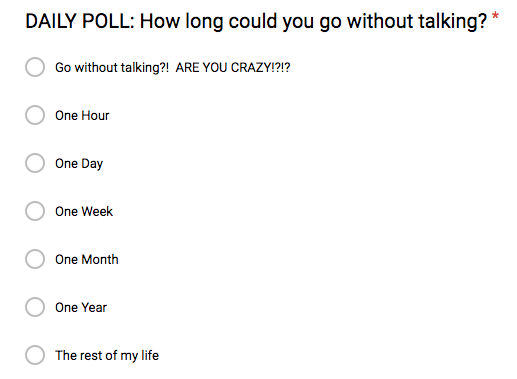This image features a webpage dedicated to a daily poll question: "How long could you go without talking?" The poll presents several options, each displayed within a clickable bubble. The options are: "Are you crazy? I can't go without talking!" (emphasized with a mix of exclamation points and question marks), followed by more measured time spans—one hour, one day, one week, one month, one year, and finally, "The rest of my life." The webpage is designed to engage users by prompting them to select the duration they believe they could remain silent, ranging from the impossibly short to the virtually unthinkable.